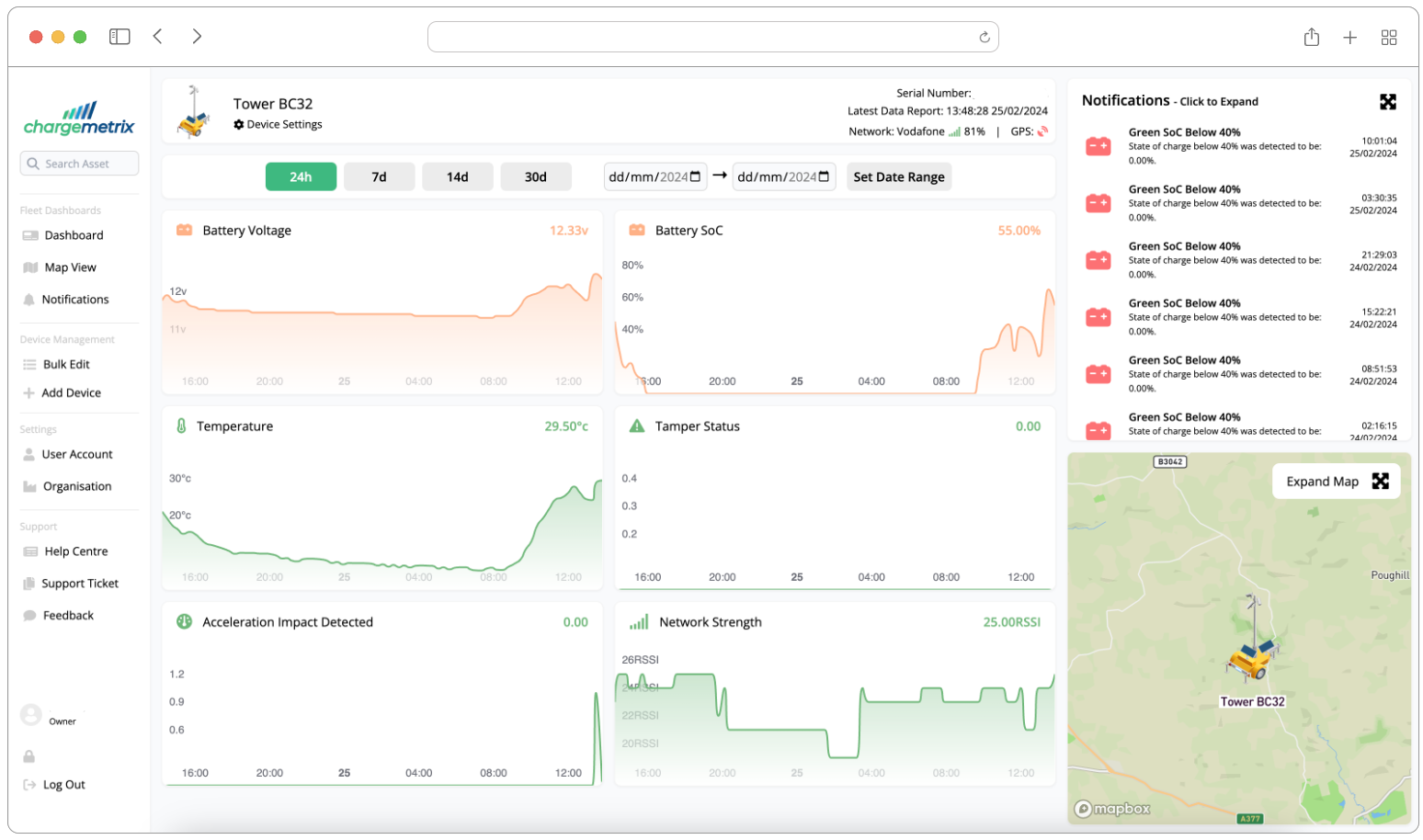This image portrays a website interface, showcasing a comprehensive and well-organized dashboard. In the top-left corner, there are three buttons—red, yellow, and green—arranged horizontally. 

Beneath these buttons, a vertical navigation menu lists various sections named: 
- Charge Metrics
- Dashboard
- Map View
- Notifications
- Bulk Edit
- Add Device
- User Account
- Operations
- Help
- Camera
- Support
- Tablet
- Feedback
- Log Out

Central to the display, detailed charts provide insights into several key metrics including battery voltage, temperature, State of Charge (SOC), and tamper status. Additional charts on the left illustrate data related to acceleration impacts, affected areas, and network strength.

On the right side of the interface, there's a Notifications button at the top. Below this, a list of different notifications keeps the user informed of recent updates and alerts.